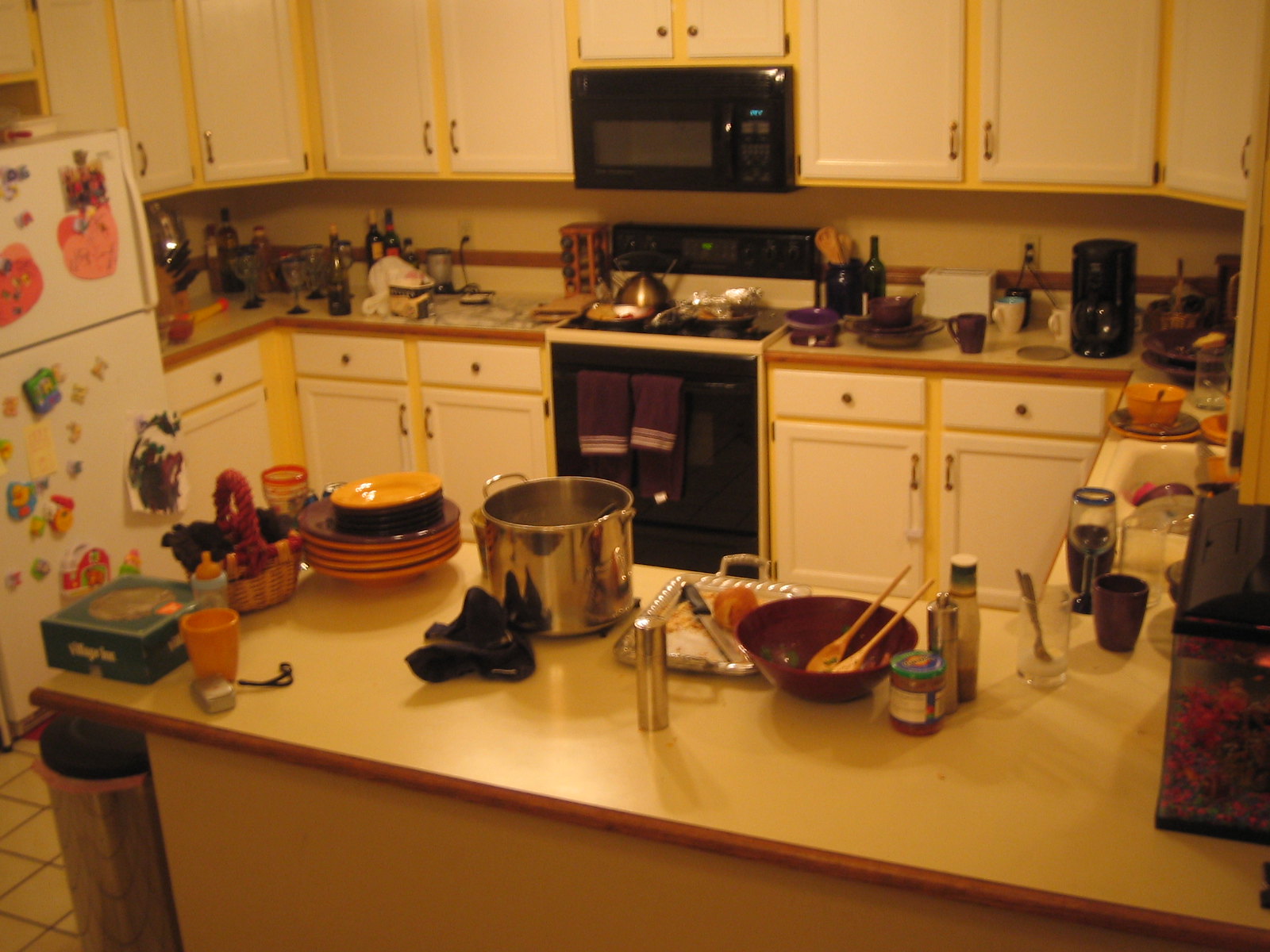A cluttered kitchen scene greets the eye, anchored by a white refrigerator with a top freezer. The refrigerator serves as a canvas for creativity, adorned entirely with pumpkin-themed artwork, colorful magnetic letters, and a watercolor painting. Moving to the counter, several bottles with cork stoppers stand alongside a sleek martini glass. An unspecified small appliance, plugged in and ready to use, occupies part of the counter space. In the corner, a spice rack is tucked away next to a pair of oven mitts.

Approaching the range, a collection of pots and pans in a striking gold color sits on the stovetop. Above, a built-in black microwave hovers, blending seamlessly with the similarly black oven below. More countertop space continues to sprawl, cluttered with various kitchenware: a green bottle, a container holding wooden spoons, three coffee cups, and a coffee pot.

The lower section of the kitchen features white cabinets set against a yellow-painted backdrop. Matching white cabinets are also found above, flanking the microwave. To the right, a sink is embedded in the counter, leading to a bar-like section, possibly designed for seating.

This extended counter holds an assortment of items: wooden bowls with spoons, food and seasoning items, a stack of clean plates, a decorative basket, a baby bottle, an orange cup, and possibly a whistle. The scene culminates with a visible trash can at the end of the counter, capturing the essence of a lived-in, functional kitchen space.